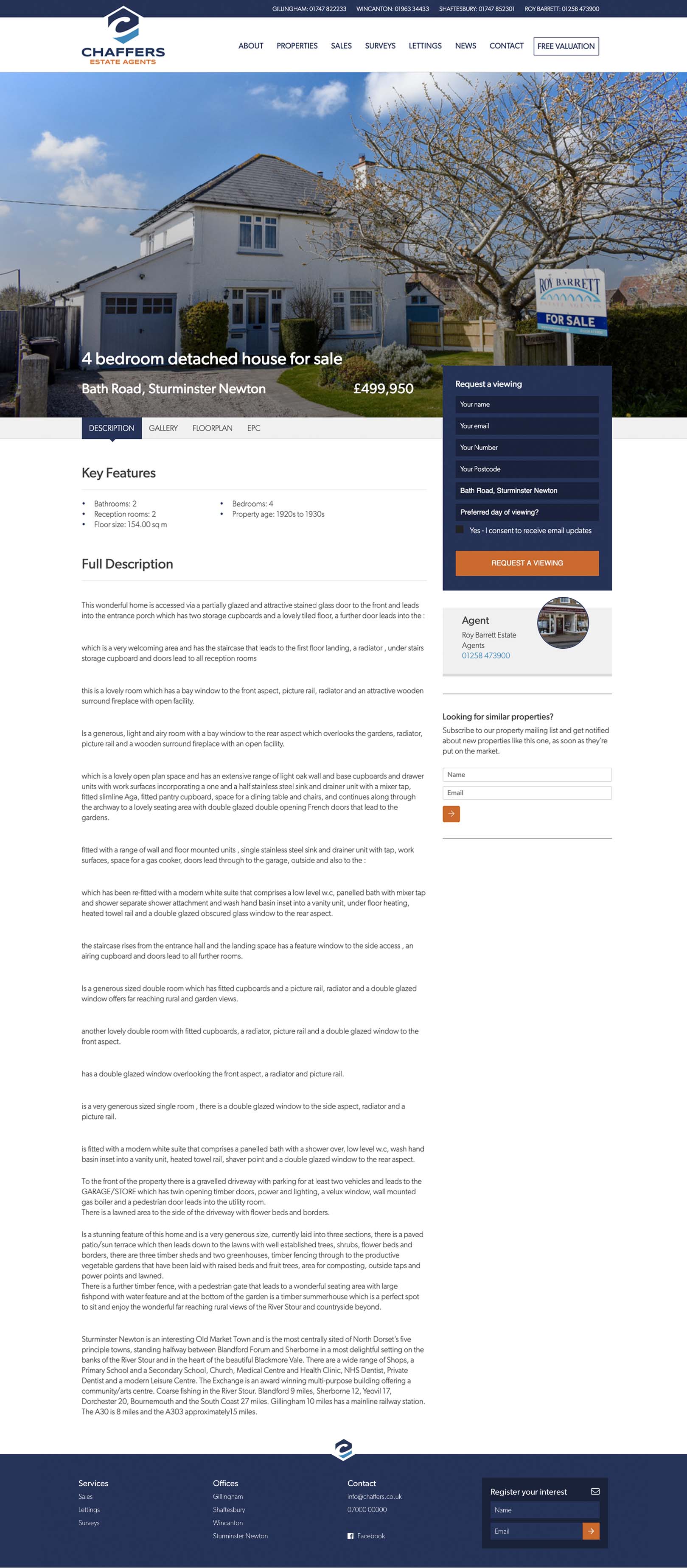This is a screenshot of a website for a real estate service called "Chaffers." The layout appears to be designed for mobile devices, as the content is displayed vertically, much like a cell phone screen. The website's header features the "Chaffers" logo, accompanied by a symbol composed of dark blue and light blue colors. Just beneath the header, there are about seven unreadable menu options, all styled in a similar shade of blue.

The main image on the page depicts a two-story white house with an attached garage. The setting appears to be a pleasant day with a blue sky and scattered white clouds. A leafless tree, possibly a cherry blossom tree, stands in front of the house, suggesting that the season could be either fall or winter. A "For Sale" sign is also present within this image, positioned on the right side.

Below the image, there is a small blue rectangle containing approximately seven or eight buttons, which are too tiny to decipher. An orange bar sits directly beneath this rectangle, carrying unreadable text as well.

Further down, the page displays a section under a blue-highlighted tab marked "Description." This section begins with a "Key Features" heading, but the specific features listed are not legible. Following this, a "Full Description" header is present, though the detailed text remains indistinct, extending significantly towards the bottom of the screen.

At the very bottom, there is a wide blue bar stretching horizontally from left to right, featuring additional clickable options in white text. Overall, the design and tiny text make the page challenging to read and navigate.